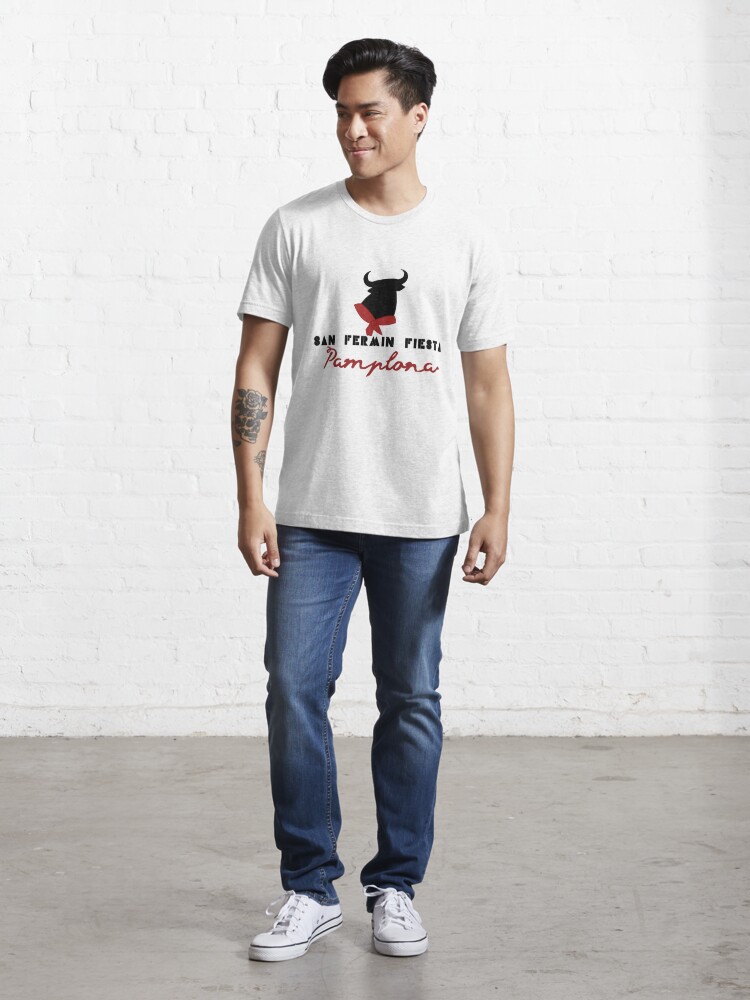In the image, a young Asian male, likely in his 20s, stands confidently against a white brick wall on a light gray cement floor dotted with some dirty skid marks. His black hair is brushed back in a neat wave, and he's turning his head slightly to the right, smiling with his eyes and eyebrows subtly mirroring his lips' closed smile. He’s wearing a white t-shirt adorned with a black bull logo that features a red scarf or bandana. The shirt reads "San Fermin Fiesta" above the logo and "Pamplona" in a red script font below it. He pairs this with slightly worn blue jeans and white sneakers. A tattoo graces his right forearm, while his arms hang casually by his sides, adding to his relaxed demeanor. His right knee is slightly bent, giving the impression of a laid-back pose.